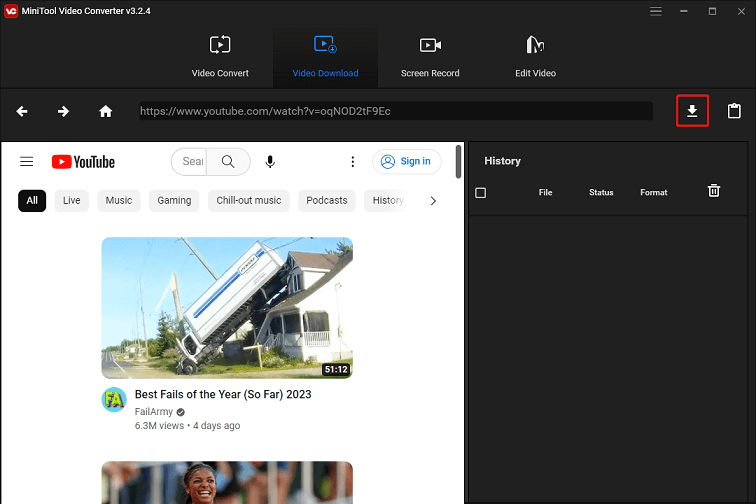Screenshot of Mini Tool Video Converter v3.2.4 Interface

The image displays the user interface of Mini Tool Video Converter v3.2.4. Prominently featured on the screen is a vibrant red box with "VC" in white text, standing for Video Converter. On the dark background, white text lists the software's functionalities: Video Converter, Video Downloader, Screen Recorder, and Edit Video. Below this text, navigation buttons including right and left arrows and a home icon can be seen.

Further down, a URL bar displays "youtube.com/watch" followed by a video identifier. A red box highlights the "Downloader" option, and alongside it, a symbol resembling a paperclip or file clip appears.

At the top of the interface, a white bar hosts the YouTube logo, a search bar, a microphone icon, and a sign-in button. Categories listed include All, Live, Music, Gaming, Chill Out Music, Podcasts, and History, with a right arrow indicating more options.

A specific video is partially visible, titled "Best Fails of the Year So Far 2023," with a duration of 51 minutes and 12 seconds. It is credited to "FailArmy," has amassed 6.3 million views, and was uploaded four days ago. The thumbnail shows a semi-truck oddly positioned on top of a house, with the truck's back end extended onto a grassy area. Another video is partially visible, though only the top edge of its thumbnail is seen.